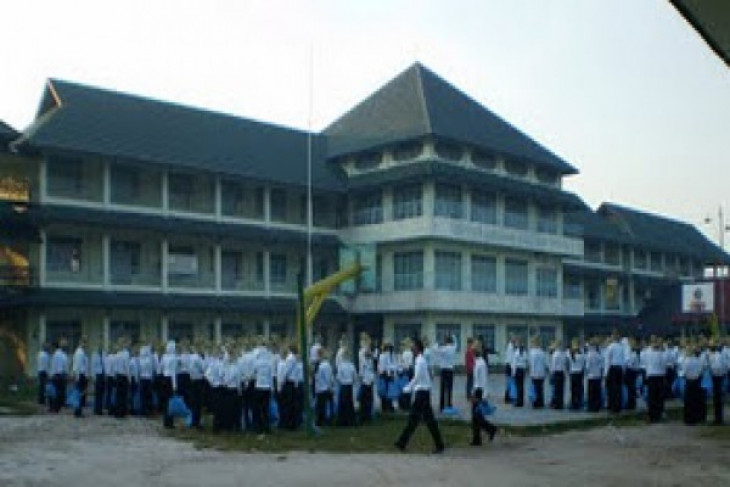The image depicts a fairly large, three-story building with a white exterior and numerous windows, accented by blue slanted roofs and a small triangular pyramid at the top, tinged gray from the sunlight on its left side. The scene takes place outdoors, where approximately 50 young students, all dressed in black pants and white shirts, are gathered near the building. The photo is slightly blurry and of low quality, resulting in muted colors across the image. The sky above is a pure white, providing a stark backdrop to the setting. 

In the foreground, the ground is tan with patches of green grass. A green pole with a yellow flag, not fully unfurled, stands slightly to the bottom left. Among the scattered individuals, two people are seen walking from right to left, with a person in red, possibly a teacher or instructor, positioned behind them. The overall arrangement appears informal yet orderly, suggesting the setting could be outside a private school or a public gathering space.